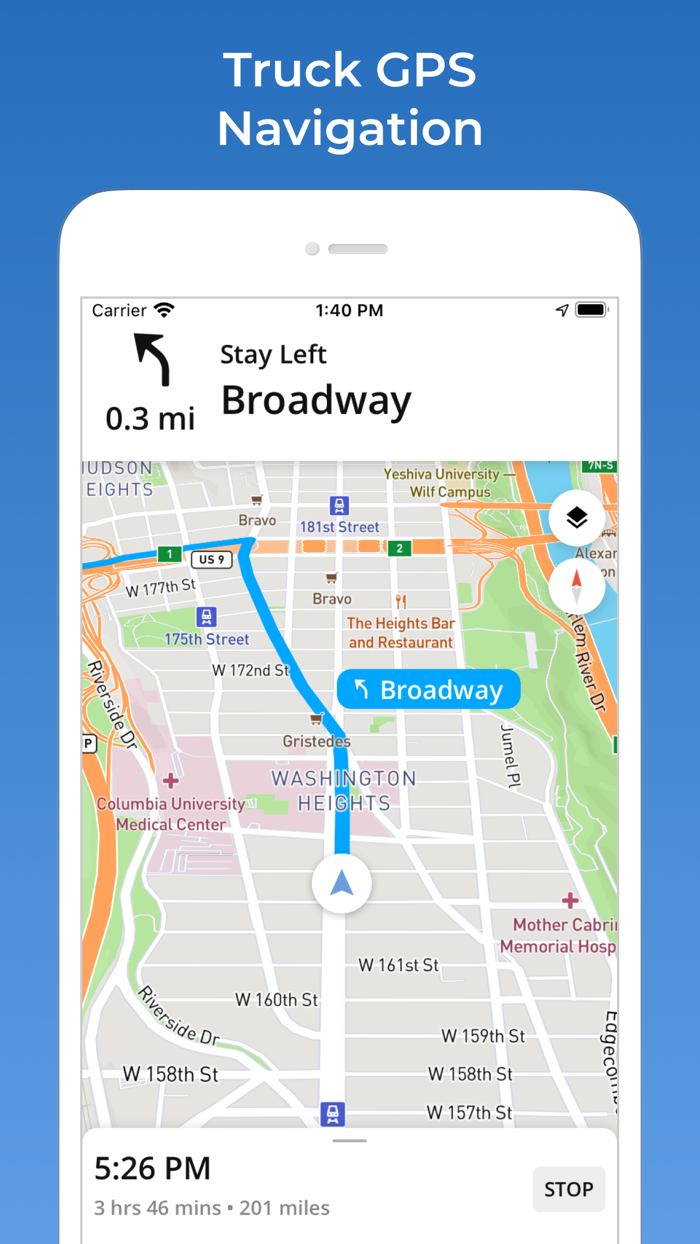In this detailed screenshot from a mobile device, we see an interface with a rectangular image that is taller than it is wide, enclosed by a blue border. At the top of the screen, in white text, it reads "Truck GPS Navigation." 

Below this heading, there appears to be a graphic representation of a smartphone display. The status bar indicates "carrier" and the time "1:40 p.m.," alongside a battery icon that shows a full charge. An arrow curving diagonally to the left is also displayed.

The main portion of the screen is dominated by a map. The navigation direction advises to "stay left on Broadway" for "0.3 mi" (miles). There is a large blue route line indicating the path, which goes upwards, diagonally to the left, and then further left.

Various points of interest and labels are visible on the map, although some text is cut off. On the top left, there is a partially visible label, "Hudson Heights." The top right features "Yeshiva University Wolf Campus." Additional landmarks include "Bravo 181st Street," "The Heights Bar and Restaurant" in the middle left, "Columbia University Medical Center" in the center, and "Mother Cambry Memorial Hosp" toward the bottom right. Numerous other street names are also present.

At the bottom of the map is a status update that reads "5:26 p.m., 3 hours 46 minutes, 201 miles stop."